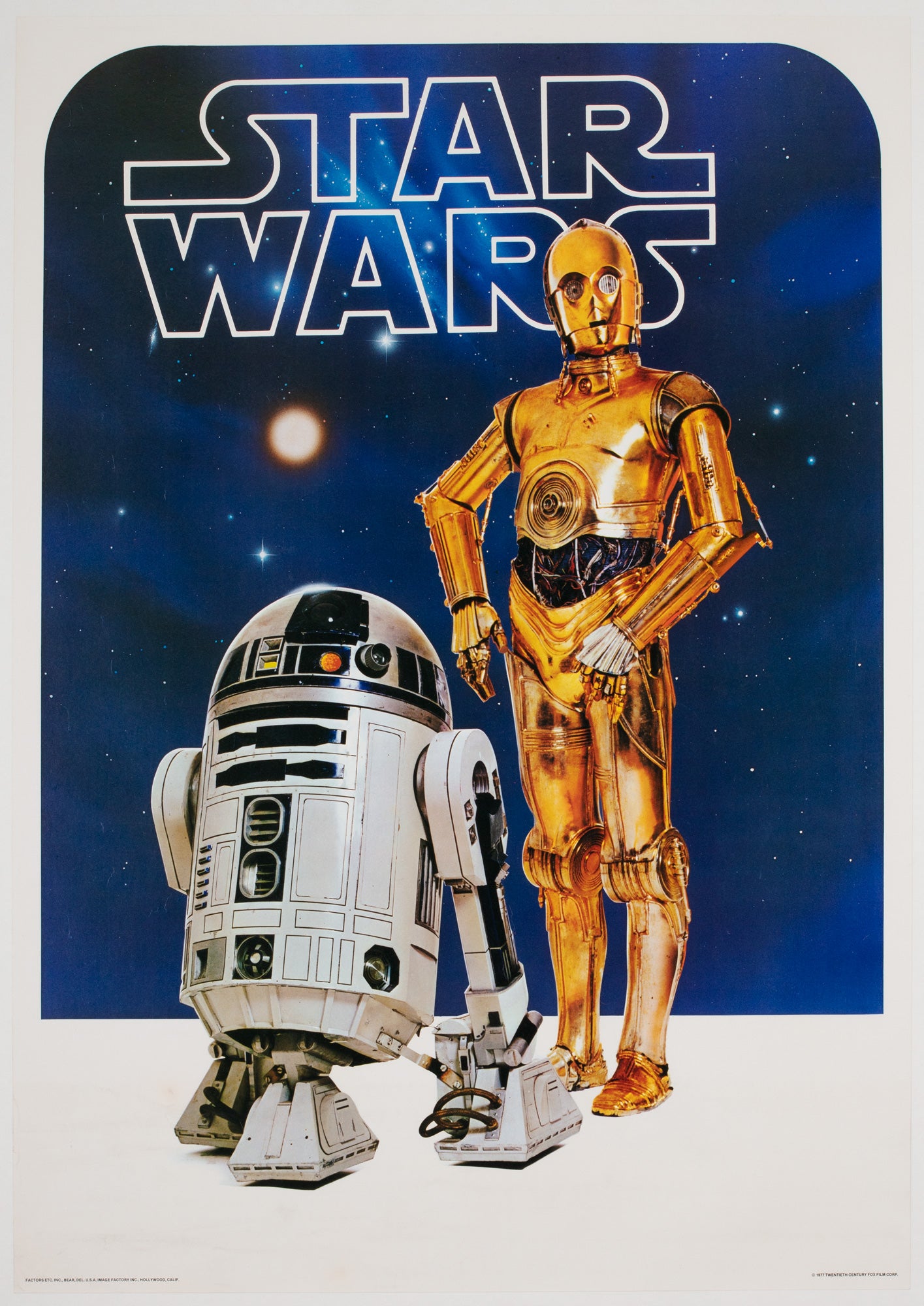This image is a poster of Star Wars, featuring a detailed nighttime scene with a navy blue sky, scattered stars, and a visible moon. At the top, in the iconic Star Wars font with white borders, the text "Star Wars" boldly stands out. Dominating the foreground are two renowned Star Wars characters, C-3PO and R2-D2. R2-D2, a small cylindrical droid with a rounded, half-sphere top and three legs, is depicted with its array of buttons and square feet. Next to it stands C-3PO, a human-like robot with a golden, hard-armored suit and a matching helmet that covers its entire head except for the eye openings. C-3PO's stiff posture with arms at its side, long jointed fingers, a big black belt, and golden shoes are clearly visible. At the bottom of the poster, there is very fine print in the corners that is too small to read.